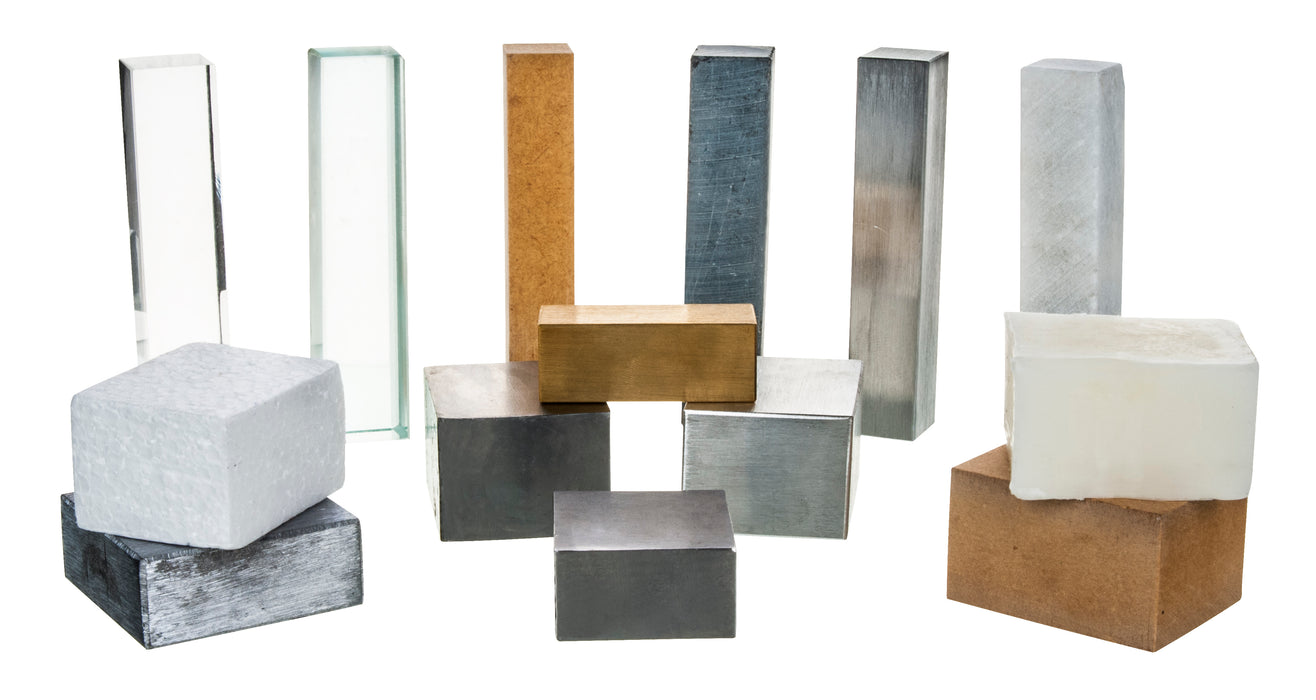This image displays an assortment of various materials, each shaped into blocks, cubes, or bars. In the foreground, there are cubes made from different substances including metal, aluminum, copper, gold, and stone. Notably, three metal cubes are positioned centrally with a wooden rectangular block bridging across two of them. Among these, one can also find cubes of wood and stone. The background features rectangular bars made of diverse materials such as clear glass, butterscotch-colored acrylic, blue acrylic, variegated blue and gray material, and white. Additional bars are crafted from wood, metals like stainless steel, and stone. The arrangement of these materials highlights a wide spectrum of colors and textures, from the metallic sheen of copper and stainless steel to the translucent quality of glass and the varied tones of stone and wood. This cohesive display captures the diversity of both material and geometric form.